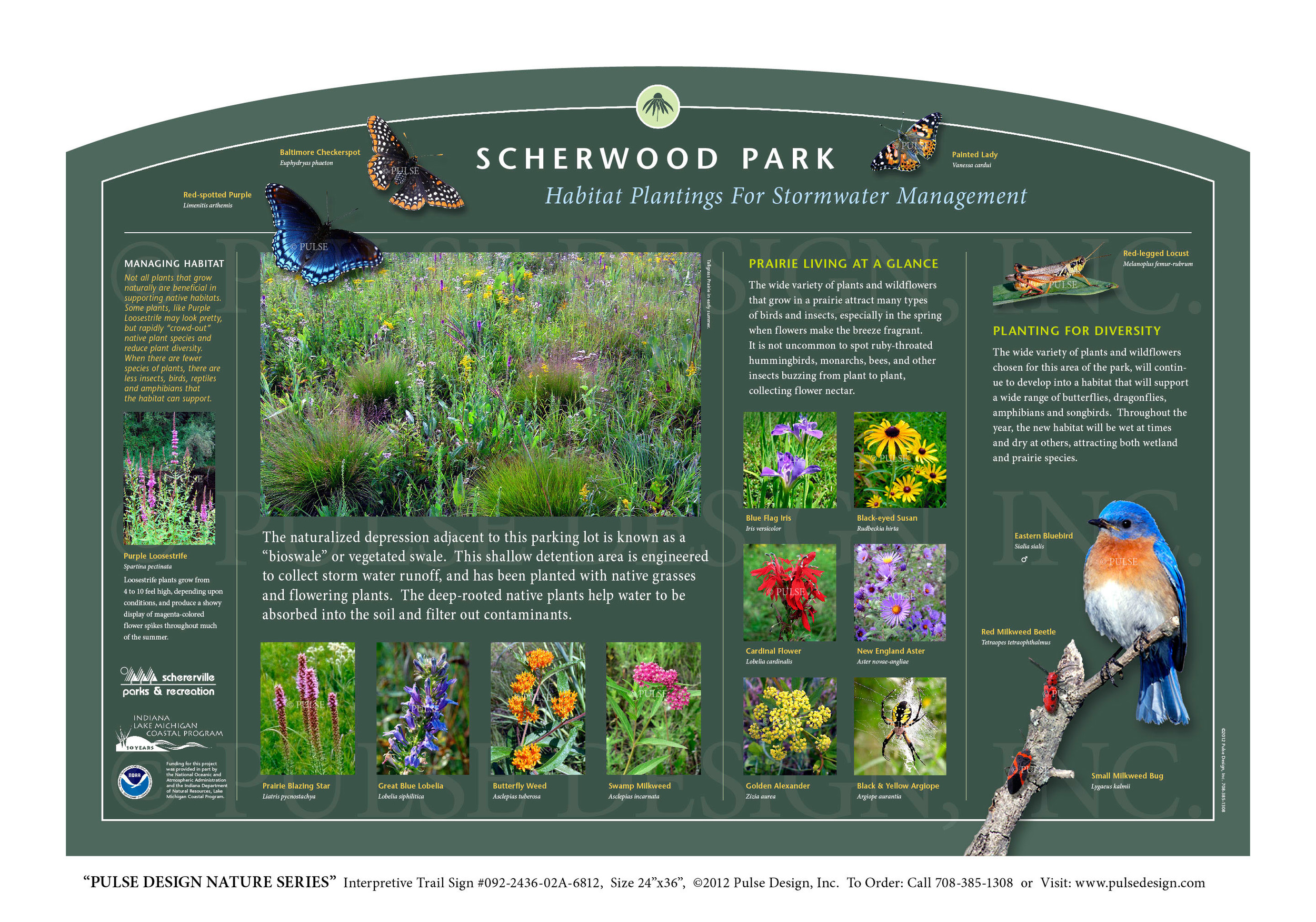The vivid image, likely a color brochure or informational chart, showcases Sherwood Park's Habitat Plantings for Stormwater Management set against a green background with a white border. Dominating the top of the image is the title "Sherwood Park Habitat Plantings for Stormwater Management" flanked by colorful butterflies, including a blue one and a pink and dark-hued one in flight, alongside another butterfly with flag-like colors. Below the title, a picture of a grassy field is displayed, followed by four diverse flower images. The right side of the image shows additional flowers, a spider, and a bird balancing on a tree branch. The text scattered around the images explains the park's mission, highlighting diverse flora and fauna, including butterflies, flowers, birds, and insects. It discusses efforts to enhance biodiversity and manage the habitat for native species and provides practical details, including contact information, website, and instructions for ordering the brochure from Pulse Design Nature Series.